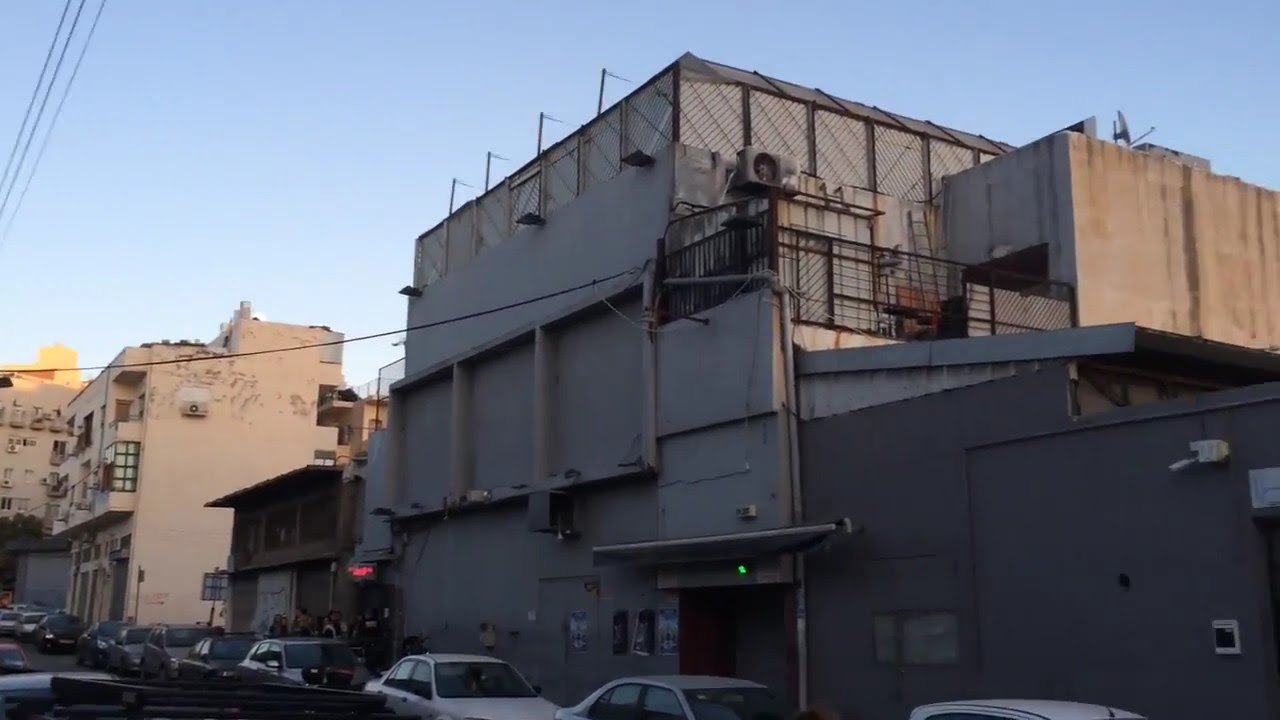This image depicts a city block on a clear, sunny day with no clouds in sight. The street is lined with a series of parked cars in front of several industrial-looking buildings. Dominating the scene, there is a massive gray building with multiple levels but no windows, giving it a stark, mechanical appearance. To the left of this building is a smaller brown structure, also windowless, which appears to meet at a junction where a group of people is gathered. Further into the background, there are two taupe-colored buildings, one positioned directly behind the other, adding depth to the composition. Power lines crisscross the scene, with one running diagonally from the upper left corner to the middle of the gray building, and others stretching across the street. Street signs are also present, contributing to the urban landscape. The entire area is sunlit, casting a bright light over the architecture and the gathered individuals, creating a vivid outdoor snapshot of an industrial part of the city.